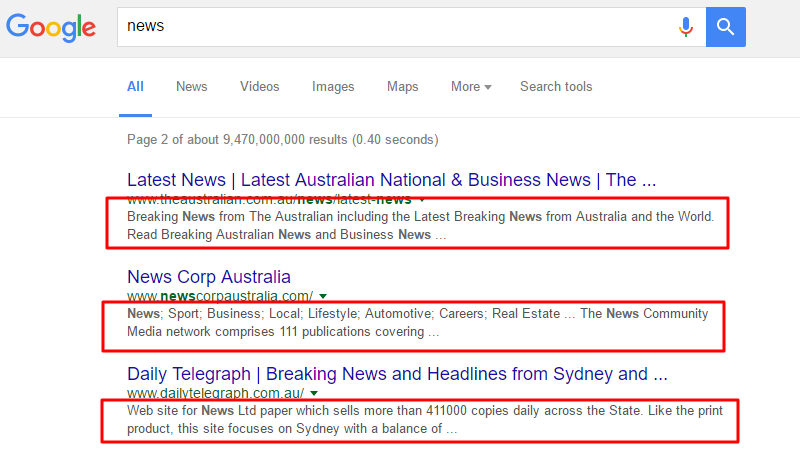This image is a detailed screen capture from a Google search result, meticulously edited to highlight specific textual information. The Google logo is prominently displayed in the top left-hand corner, signifying the source of the search. At the center, the search bar shows the query "news" with a microphone icon and a search button icon to its right.

Directly below the search bar are tabs for filtering search results, with "All" being the selected option. Adjacent tabs include "News," "Videos," "Images," "Maps," and a "More" drop-down button. Additionally, a "Search tools" option is visible. The search results summary reads, "Page 2 of about 947,000,000 results (0.4 seconds)."

A section titled "Latest news" follows, listing headlines underlined by red boxes. The first red box emphasizes the text: "Latest Australian national and business news," with a notable highlight of "Breaking news from the Australian, including the latest breaking news from Australia and the world. Read breaking Australian news and business news…"

Further down, News Corp Australia is mentioned, with another red box underscoring "News, sports, business, local, lifestyle, automotive, careers, real estate…" highlighting the broad spectrum of news it covers. The accompanying note adds, "The news community media network comprises 111 publications covering…"

Lastly, the Daily Telegraph is featured with a red box focusing on, "Website for news, LTD paper which sells more than 411,000 copies daily across the state. Like the print product, this site focuses on Sydney with a balance of…"

This detailed and annotated screen capture effectively highlights significant text within a Google search result page, guiding the viewer's attention precisely to the intended information.